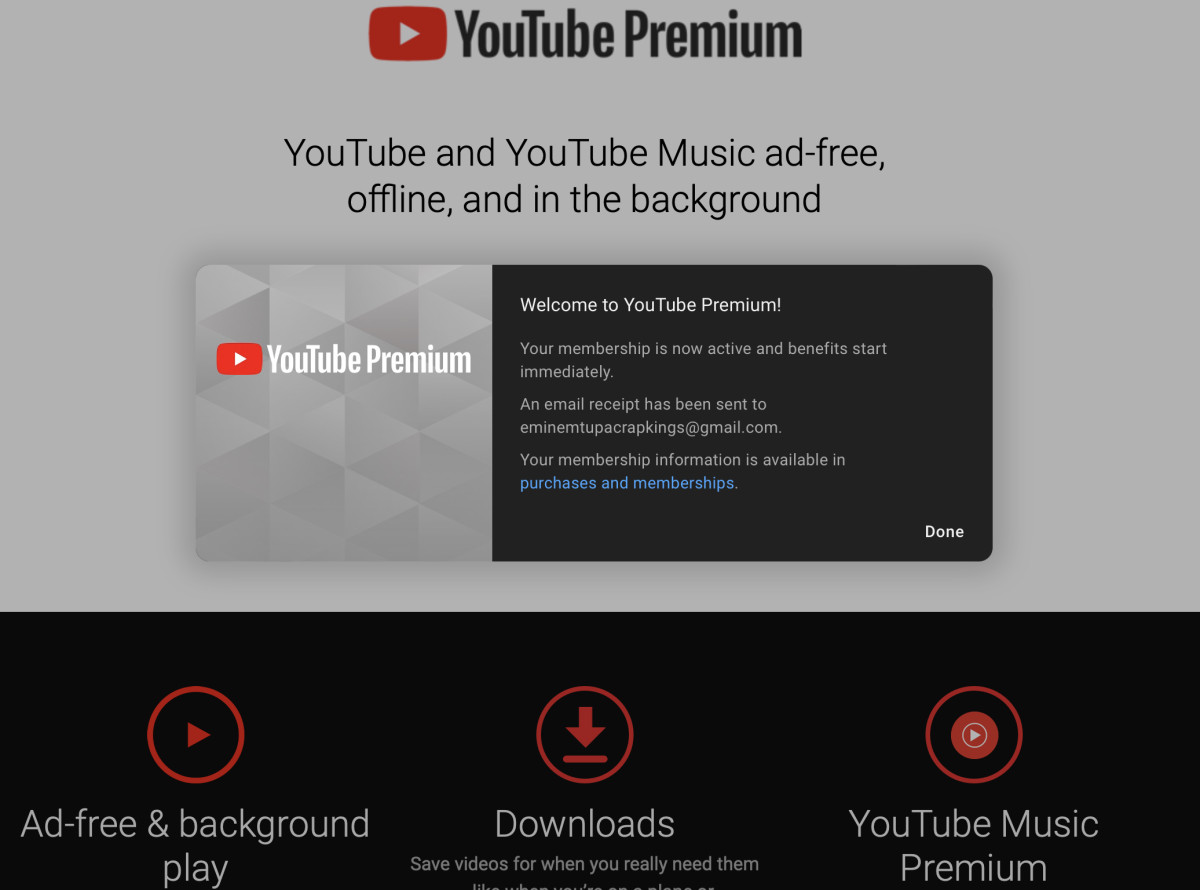A screenshot of a YouTube Premium subscription confirmation page. At the top of the image is a large gray box displaying the YouTube Premium logo, which consists of a red rectangular box with a silver play button icon and the words "YouTube Premium" in black. Below the logo, the text reads "YouTube and YouTube Music ad-free, offline, and in the background."

Beneath this, another gray box contains the welcoming text: "Welcome to YouTube Premium. Your membership is now active and benefits start immediately. An email receipt has been sent to EminemTupacRapKings@gmail.com. Your membership information is available in 'Purchases and memberships'." At the bottom of this box, there is a "Done" button for users to complete the process.

Underneath this main section, a black bar features three options, each accompanied by a red circle with a corresponding icon in the center. The options are, from left to right: 
1. "Ad-free and background play" with a play button icon.
2. "Downloads: Save videos for when you really need them" with a download icon.
3. "YouTube Music Premium" with a play button encircled by a ring.

The overall design is clean and clearly outlines the benefits of the YouTube Premium membership, ensuring the user is informed and ready to enjoy their new subscription features.